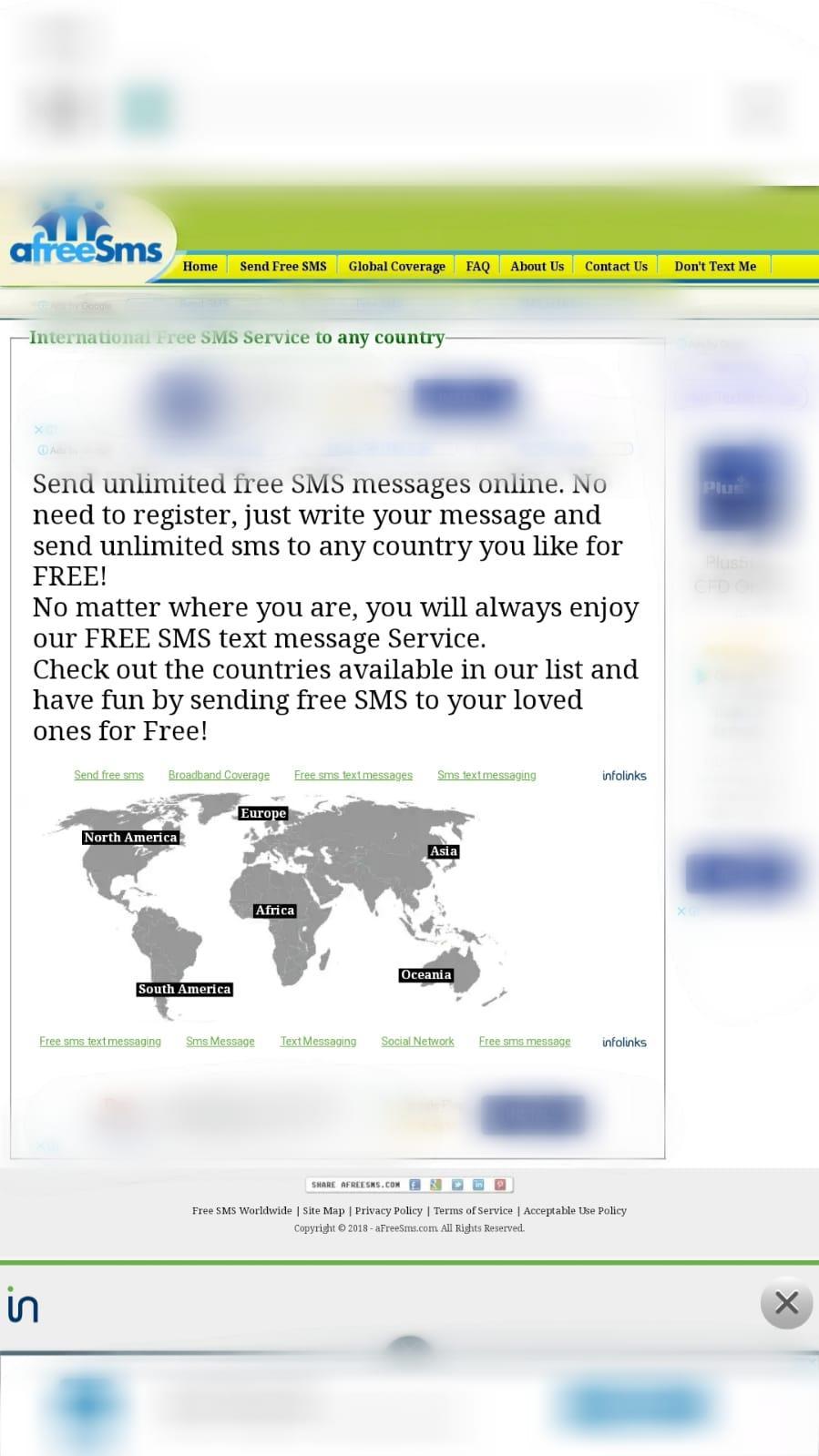The image portrays a web page offering a free SMS messaging service. In the top left corner, the text "free SMS" is prominently displayed as a single word. This indicates that users can send SMS messages online for no charge. To the right, an options panel features clickable yellow rectangles, providing access to various functionalities.

Centered within the page, grey text boasts the service’s benefits: "Send unlimited free SMS messages online. No need to register, just write your message and send unlimited SMS to any country you like for free! No matter where you are, you will always enjoy our free SMS text messages service. Check out the countries available in our list and have fun by sending free SMS to your loved ones for free."

Beneath this text, a map of the world is displayed, showcasing the continents shaded in grey. The map gives a visual representation of the service’s global reach, although individual countries are not delineated. The blurred section of the webpage adds an element of mystery, partially obscuring the full scope of the service options available.